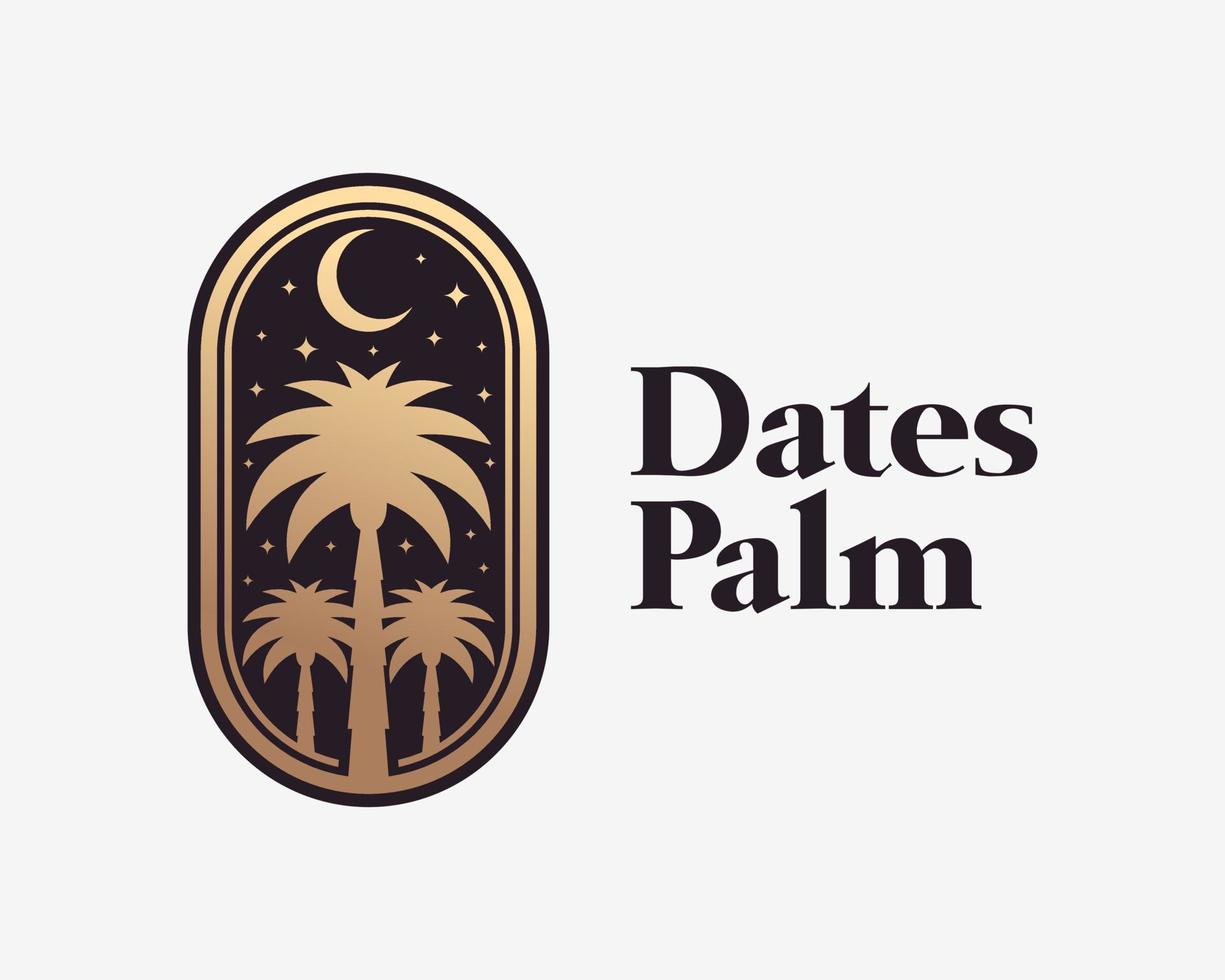The image appears to be a logo set against a very light gray background, featuring a prominent black text that reads "DATES" above "PALM" on the right side. To the left of the text is an oval-shaped, gold-bordered emblem. Inside the oval, a larger central palm tree flanked by two smaller palm trees, all in gold or brass, form the focal point. Above the central palm tree, a gold crescent moon is set amidst a backdrop of 17 scattered gold stars. These elements together create a balanced and intricate design, surrounded by a gold oval with a black stripe and then an additional black external border. The overall presentation makes use of simple but bold visuals to convey a distinctive and memorable logo, possibly for a brand or product associated with palm dates.